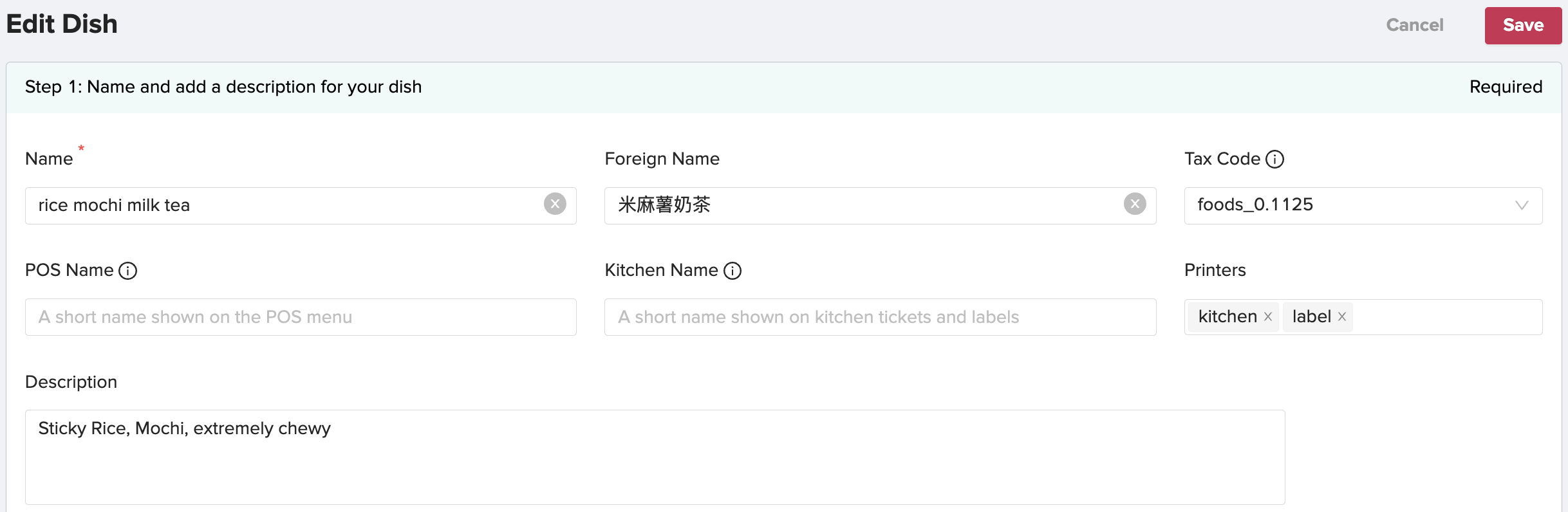This is a partial screenshot of a web page displayed on a computer monitor. At the top of the page, there is a black banner with the text "Edit Dish." On the far right of this banner, there are two buttons: a "Cancel" button and a red "Save" button.

Below the banner is a sky blue section labeled "Step One: Name and added description for your dish," with the word "Required" indicated on the right side. Beneath this section are input fields where users can enter the name of the dish and additional details. These fields include an area for "Name" and another labeled "Foreign Name," both featuring small "x" icons for clearing the input.

Adjacent to these fields, there is a "Tax Code" label accompanied by an information icon (a circled "i"), under which is a dropdown menu displaying the text "foods_0.1125." 

Further down, there is another set of input fields: one for "POS Name," also accompanied by an information icon, and another box titled "Kitchen Name." Descriptive text under "Kitchen Name" states "Short name shown on kitchen tickets and labels." To the right is a section titled "Printers" with tabs labeled "Kitchen" and "Label," both of which can be expanded or collapsed.

Below the "Printers" section, there is a text area labeled "Description," pre-filled with the text "Sticky rice mochi, extremely chewy."

The page allows users to edit and save information about a dish in a restaurant's digital menu, with all necessary fields and information clearly outlined for efficient editing and updating.